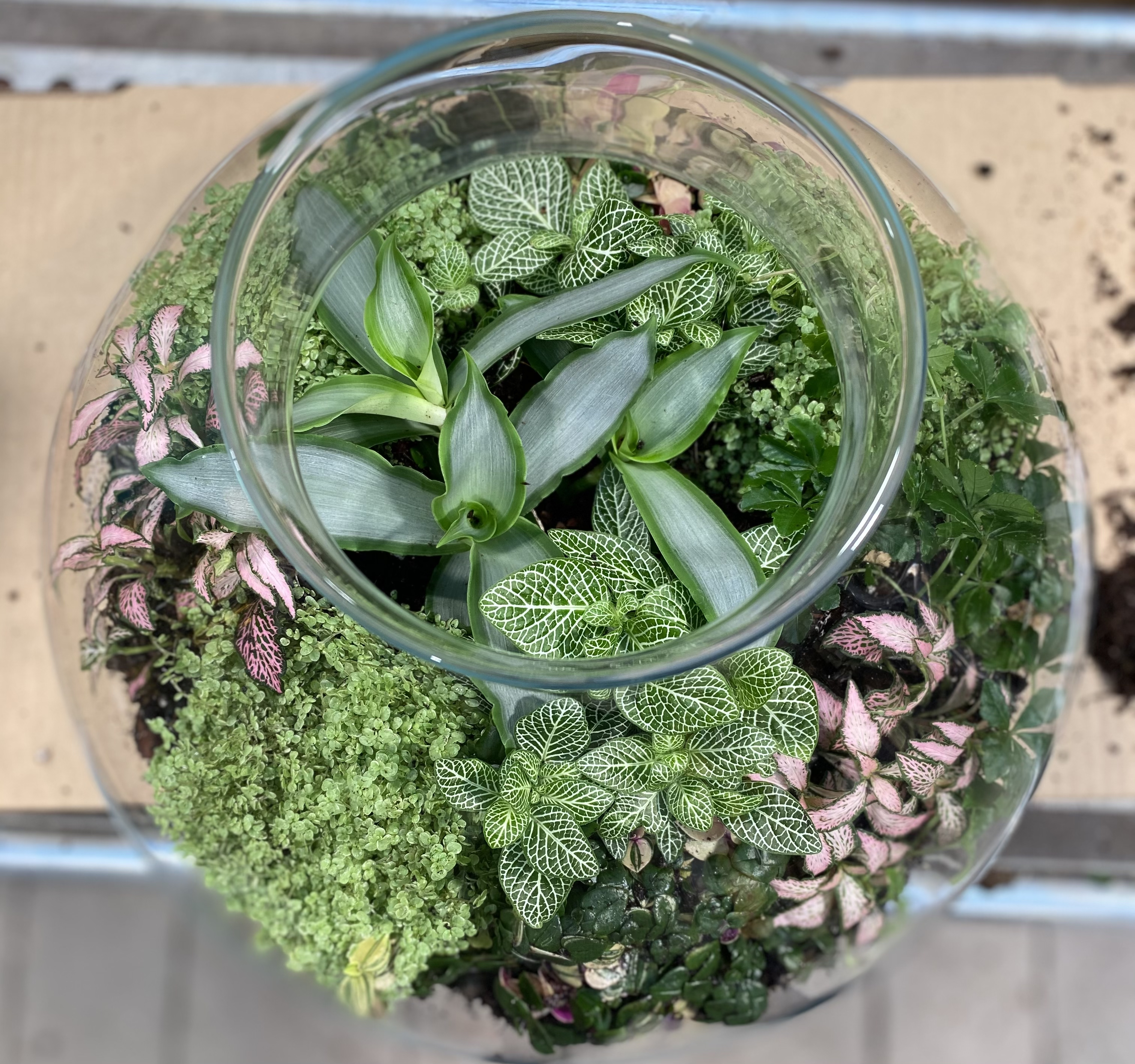The image depicts a realistic and visually appealing photograph of a round glass fishbowl, which takes up the majority of the frame. Inside the clear fishbowl, a variety of greenery is flourishing, including larger and smaller leaves with varying shades of green—some vibrant, some paler, and others with distinct shapes like sharp or wavy edges. Among the greenery, there's also a striking plant with pinkish-reddish leaves edged in dark green. The bowl is resting on a concrete ledge that appears to be on top of a steel grate placed on a wooden floor, as the different wood panels, though slightly blurry, can be seen. The arrangement suggests that the bowl was freshly filled with soil and plants, adding to its lush and well-kept appearance.